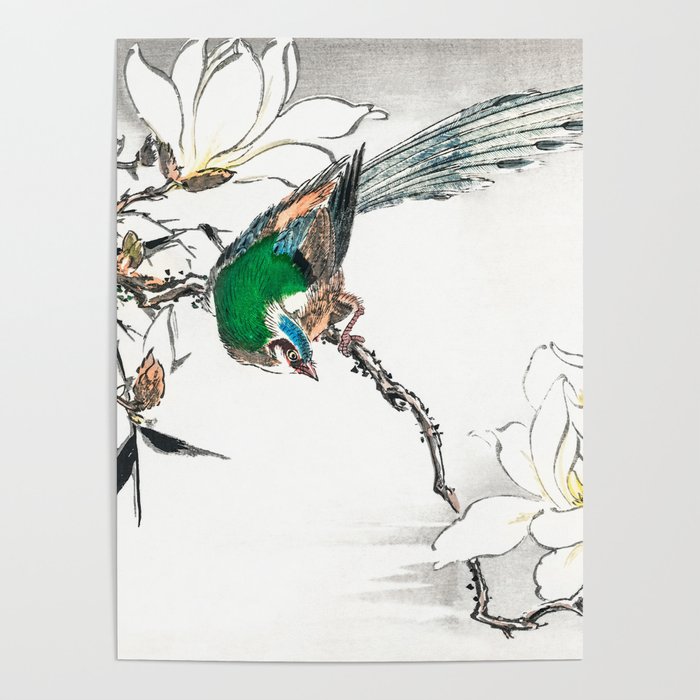This image is of a Japanese-style watercolor drawing depicting a brightly colored bird perched on a twisted branch, staring intently at a white lotus flower. The bird, identified as a young peacock, showcases vibrant green feathers on its back and neck, a prominent blue mark extending from its beak to the back of its head, and multicolored wing and tail feathers in shades of black, blue, and light brown. Its tiny pink feet grasp the brown branch, which also holds budding white lotus blossoms. The scene is set against a mostly white background with subtle gray shading at the top, enhancing the floating appearance of the artwork. The composition is detailed, with no accompanying text, capturing a delicate and intricate snapshot of nature.